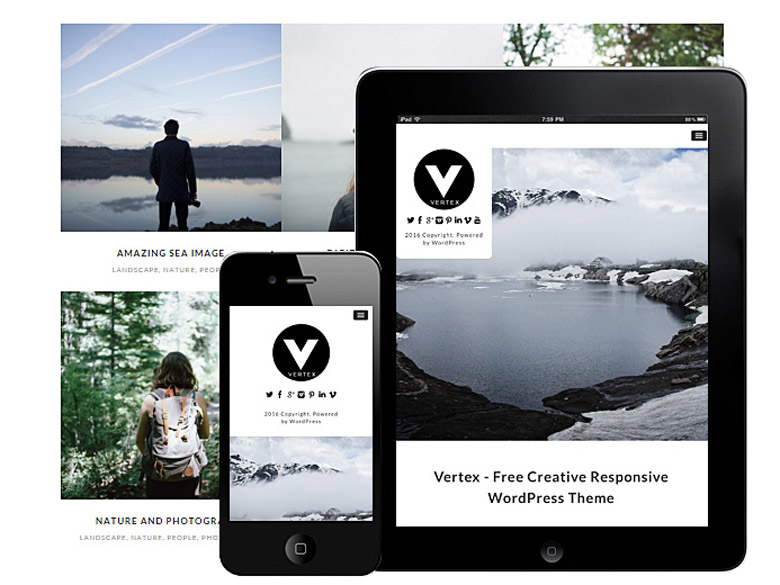The image appears to be a promotional advertisement for a WordPress theme called "Vortex," designed for showcasing creative content. The scene features multiple electronic devices, including a black iPhone and a black iPad, both prominently displaying the same serene image of a fog-covered lake with a distant snow-capped mountain range and clouds overhead. The Vortex logo is visible on the devices, and the iPad screen specifically highlights the text: "Vortex Free Creative Response WordPress Theme," suggesting the theme's compatibility with both phones and tablets.

In the background behind the iPhone, there's a photo of a girl walking through a forest, equipped with a backpack and wearing a sleeveless shirt, embodying the theme of "nature and photography." This indicates the theme's capability of incorporating landscape and adventure imagery.

Above the forest image, there is another picture showing a man gazing at a expansive cloud-filled sky over the ocean, captioned with "Amazing Sea Images," hinting at the WordPress theme's ability to beautifully showcase sea and sky photography. The overall layout suggests a versatile WordPress theme ideal for creatively displaying nature and landscape photography across various digital devices.